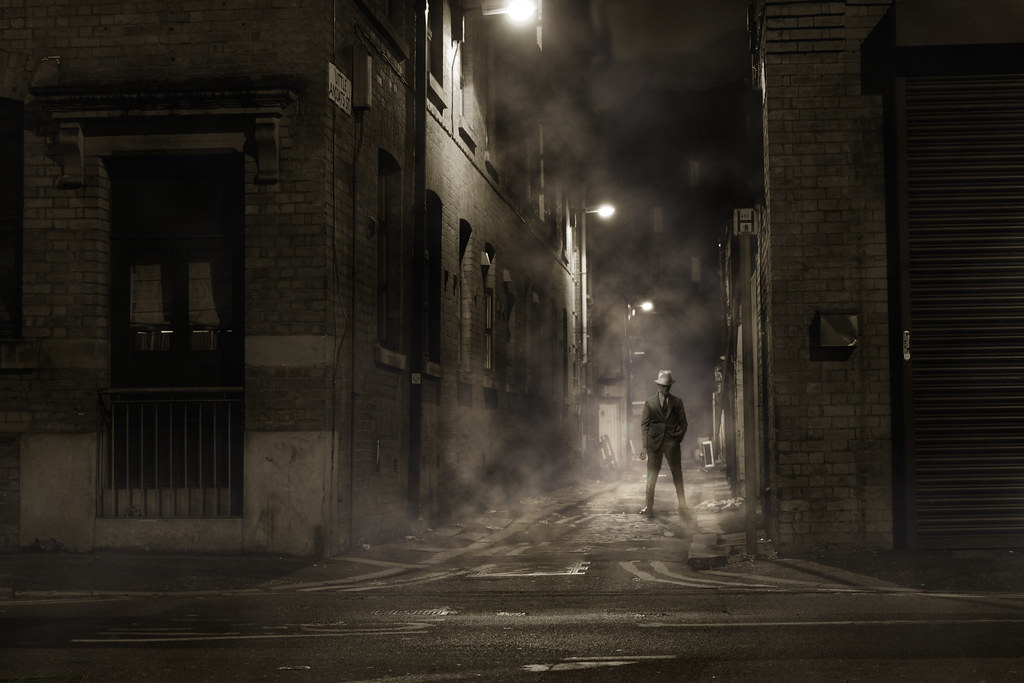In this mesmerizing, noir-inspired nighttime scene, we observe a solitary man standing in a dark, fog-enshrouded alley. Dressed in a meticulous outfit comprising a gray double-breasted suit, a black tie, and a fedora, his left hand casually rests in his pocket, adding an air of mysterious intent—possibly even threatening. The alley, paved with asphalt, is flanked by towering, old reddish-brown brick buildings adorned with multiple windows and occasional railings. Some parts of these structures resemble garage fronts, while a barred doorway is also visible on the left. Illuminated by three scattered streetlights, the scene is further accentuated by swirling smoke and dense fog, creating an ominous and gloomy atmosphere devoid of any vehicles or other people.